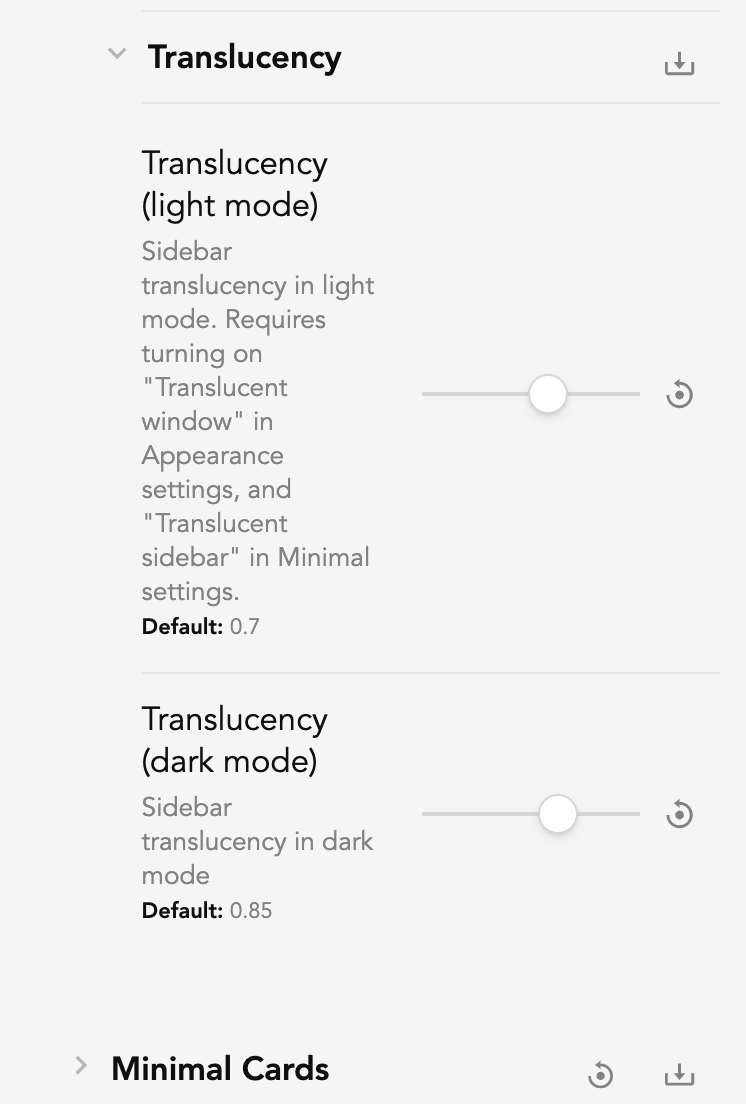This is an image of a cell phone's settings screen displayed in a vertical rectangle format. The background is a subtle gray, providing a neutral backdrop for the black and gray text. 

At the top of the screen, there is a section labeled "Translucency," accompanied by a downward-facing arrow indicating expandable options within this category. To the right of this label is a download icon, suggesting that additional resources or settings may be available for download.

Beneath the "Translucency" header, the first setting is "Translucency Light Mode." A brief instruction is provided, explaining that enabling the light mode requires activating translucent window functionality in appearance settings and translucent sidebar in minimal settings. The default translucency level for light mode is set at 0.7. Adjacent to this descriptive text is a slider bar illustrated with a large circle on a gray line, allowing users to adjust the translucency level to their preference. To the right of the slider, there is a return button that permits users to revert to the previously saved setting for light mode.

The next section addresses "Translucency Dark Mode." Similar to the light mode, this setting includes a brief description informing users that the default translucency level for dark mode is 0.85. This section also features a slider bar, enabling adjustments to the translucency level, with an accompanying return button for restoring the previous setting.

Below the translucency settings, there is an option labeled "Minimal Cards" with a right-facing arrow, indicating that selecting this option will lead to additional settings or options. This section also includes a return function and a download function, allowing users to navigate back to prior settings or download further options.

The overall layout provides a clear and detailed interface for adjusting translucency settings on the device, with easily recognizable icons and functional buttons for user convenience.